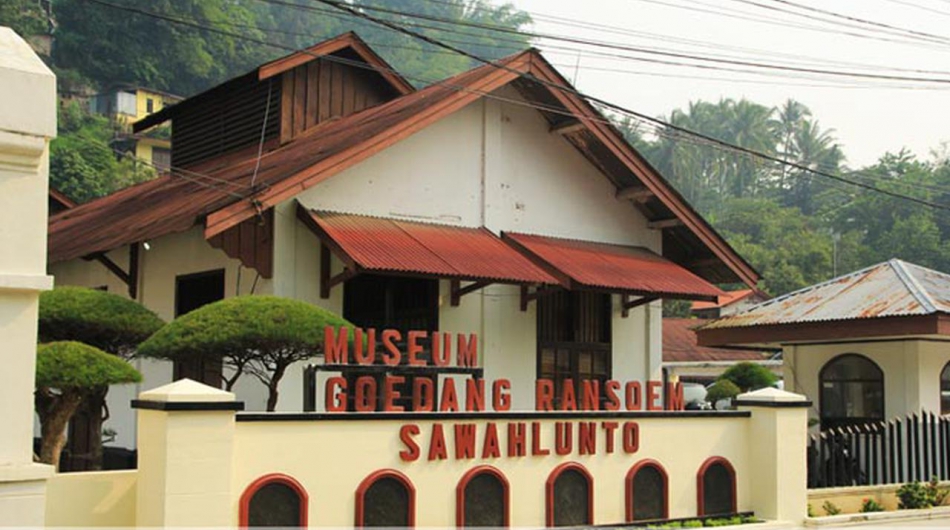This photograph depicts the front of a museum identified by a sign in red letters that reads "Museum Goedang Ransom Soehlunto" with "SAWAHLUNTO" written in all caps beneath it. The building itself is cream-colored with a distinctive red gabled roof and two red awnings adorning the front. To the left, three flat topiary trees and manicured shrubbery along a small stucco wall enhance the setting. In the background, a lush hillside with green trees and a glimpse of gray sky partially obscured by electrical wires can be seen. A small, rusty tin-roofed building is visible to the right, adding to the quaint neighborhood charm.